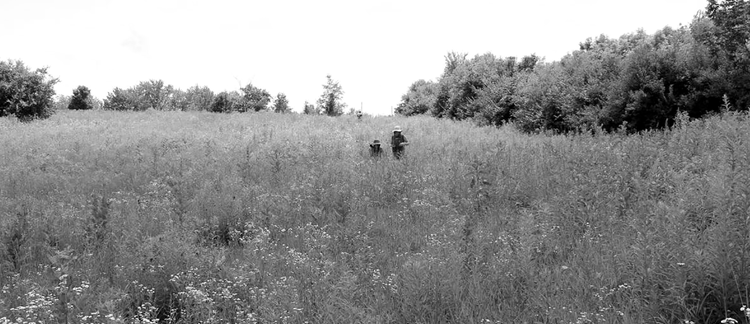This black-and-white photograph captures a vast, open field overgrown with tall grass and dotted with wildflowers. The field is bordered by a tree line extending from the left side of the photograph to the right, with a dense forest area on the right and sparser trees on the left. At the center of the image, two people can be seen walking through the tall plants, wearing hats and older clothing, suggesting that they might be elderly or that the photo could be an antique or recreation. There appears to be a third figure further back in the distance, but the details are too indistinct to be certain. The bright sky adds contrast to the scene, highlighting the expansive and slightly untamed nature of the field.